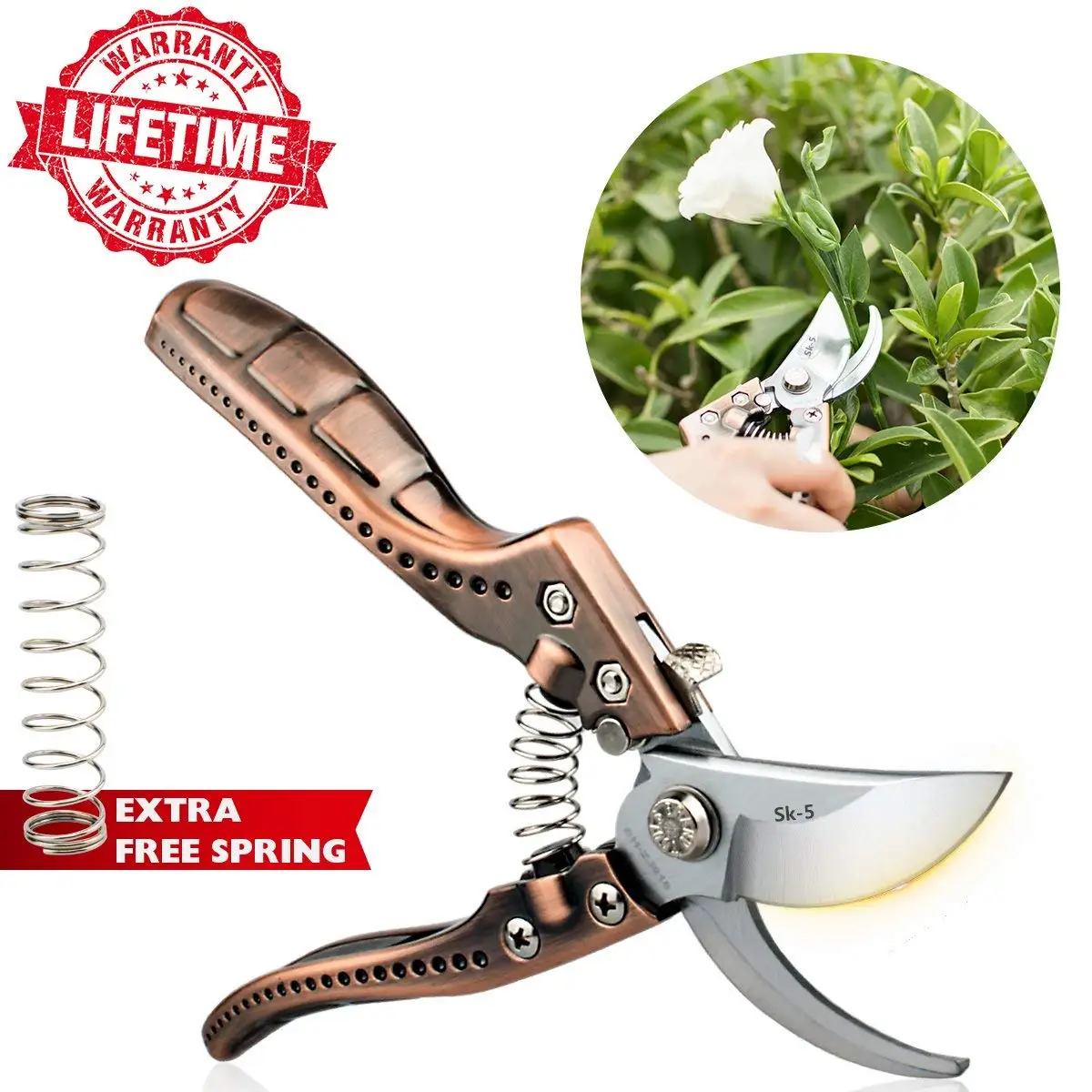This image highlights a set of high-quality, metal pruning shears prominently placed at the center, set against a white background. The shears feature a brass-colored handle adorned with four square patterns on the top handle and some engraved circles along the length, providing both functionality and an elegant design. The blades are silver with a chromed rivet in between, indicative of durability. A visible safety latch is situated on the top handle, and the shears are held open by a sturdy center spring. Notably, a text block to the left of the shears boasts an additional free spring included with the purchase.

In the upper left corner of the image, a red-and-white "Lifetime Warranty" label assures buyers of the product’s lasting quality. A smaller inset in the top right corner shows the shears in action, with a close-up shot of a hand using them to cut a white flower, highlighting their precision and utility in real-life usage. Additionally, the model identifier "SK5" is subtly marked on the top blade, indicating the specific type of steel used.

Overall, this meticulously detailed product advertisement underscores the durability, utility, and refined design of these garden shears, making it a compelling buy for any gardener.